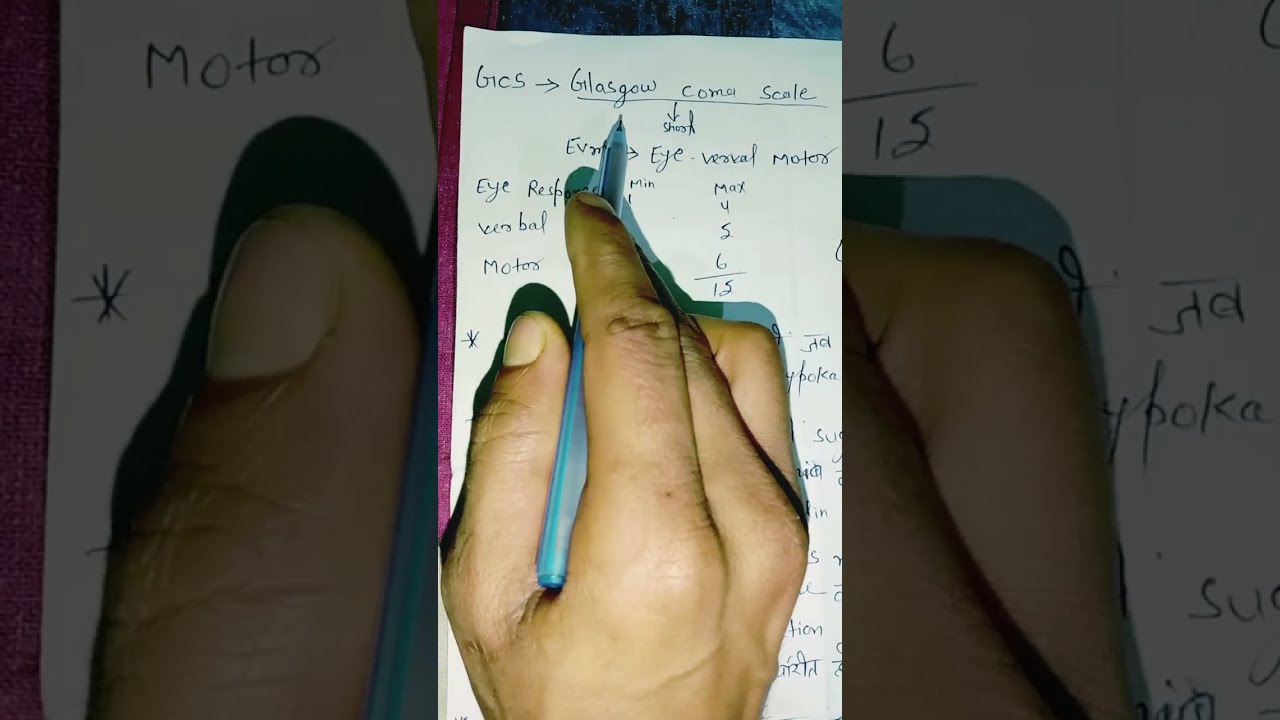In this high-angle close-up shot, a person's hand with an olive complexion is captured mid-action while writing on a piece of white paper. The hand, holding a solid blue ink pen between the thumb and index finger, dominates the image and points towards the word "Glasgow." Several handwritten notations can be seen on the paper, suggesting a detailed assessment or analysis. The text includes phrases like "GC5" with an arrow pointing forward, 'Glasgow, scale,' which is underlined, and notation like "I response, verbal, motor," along with numerical values "4, 5, 6, 15." The presence of arrows, formulas, and medical terminology indicates that the note might be related to a medical or scientific context, possibly from a doctor. The lighting above illuminates the scene, accentuating the pen and the hand's action while casting shadows over parts of the text, some of which remain obscured under the hand. The intricate details and complex notations suggest a professional or scientific task in progress.